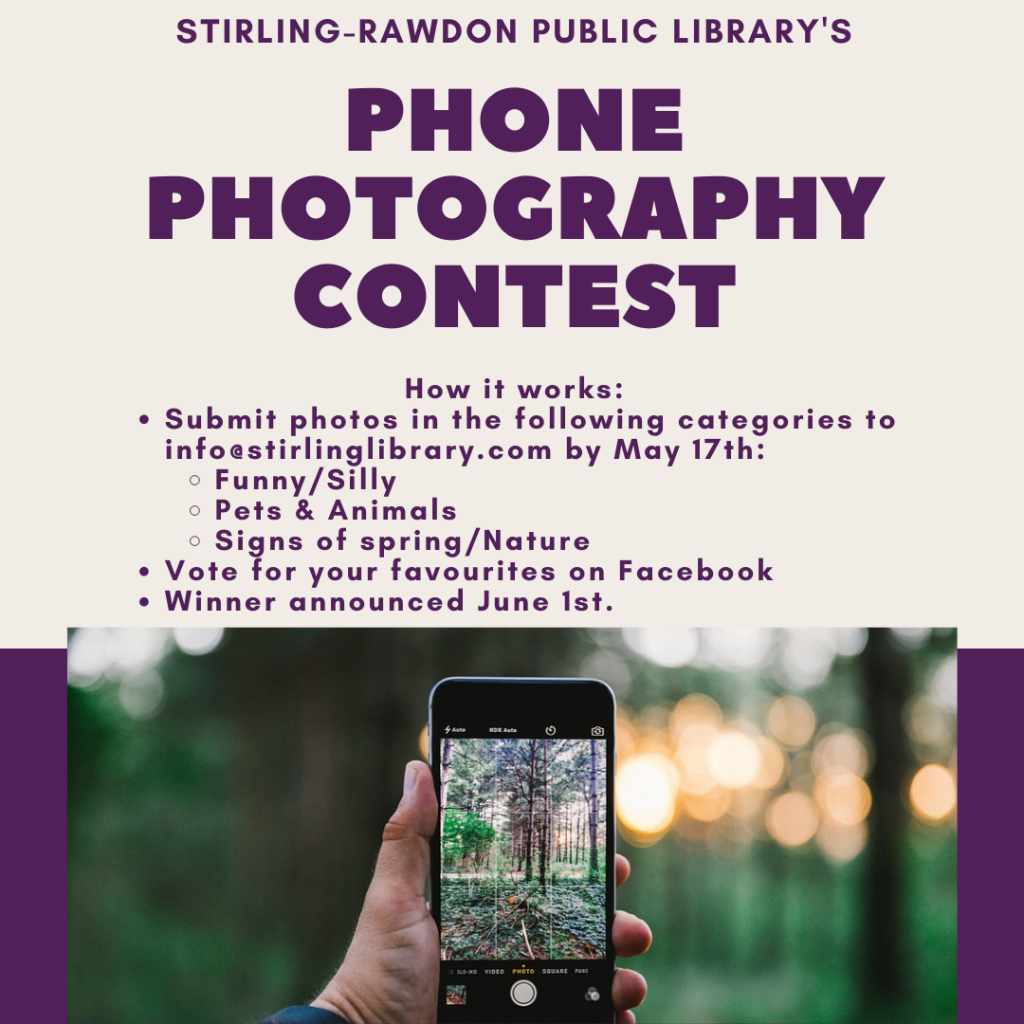The image is an advertisement for the Sterling Rawdon Public Libraries Phone Photography Contest. The top two-thirds of the image features an off-white background with purple text. At the very top, it reads "Sterling Rawdon Public Libraries Phone Photography Contest" in large, bold print. Below that, detailed instructions are provided in smaller text: "Submit photos in the following categories to info@sterlinglibrary.com by May 17th: Funny/Silly, Pets and Animals, Signs of Spring/Nature. Vote for your favorites on Facebook. Winner announced June 1st."

Occupying the bottom section is a color photograph of a white person's left hand holding a smartphone, which displays an image of a forest scene. The phone shows tall trees and possibly some vines, suggesting the photo was taken in a wooded area. The background behind the phone is blurred, likely showing the same forest with large, out-of-focus orange spots that might hint at either sunlight filtering through the trees or a setting sun. The overall image combines the detailed contest information with an illustrative photo that highlights the theme of capturing nature through phone photography.